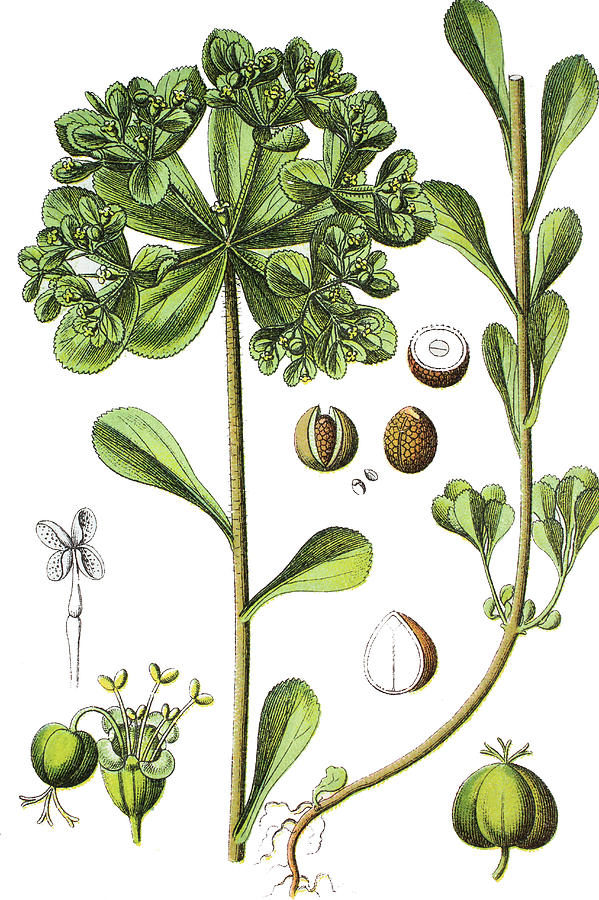This detailed piece features a vertically rectangular, multi-color artistic interpretation of various green plants against a pure white background. At the center, one plant is depicted with a thin cylindrical stalk adorned with oval-shaped green leaves and a cluster of small yellow blossoms at the top. Several of the illustrations, reminiscent of a detailed scientific diagram, showcase different aspects of the plants. To the left, there is a black and white cartoon-style diagram of a plant that includes seeds, some of which are whole while others are cut to reveal a rough exterior and white interior. Scattered around the main images are additional smaller illustrations, including close-ups of plant stalks and root systems, the latter of which are small and not very extensive. The seeds appear brownish-orange with white interiors.